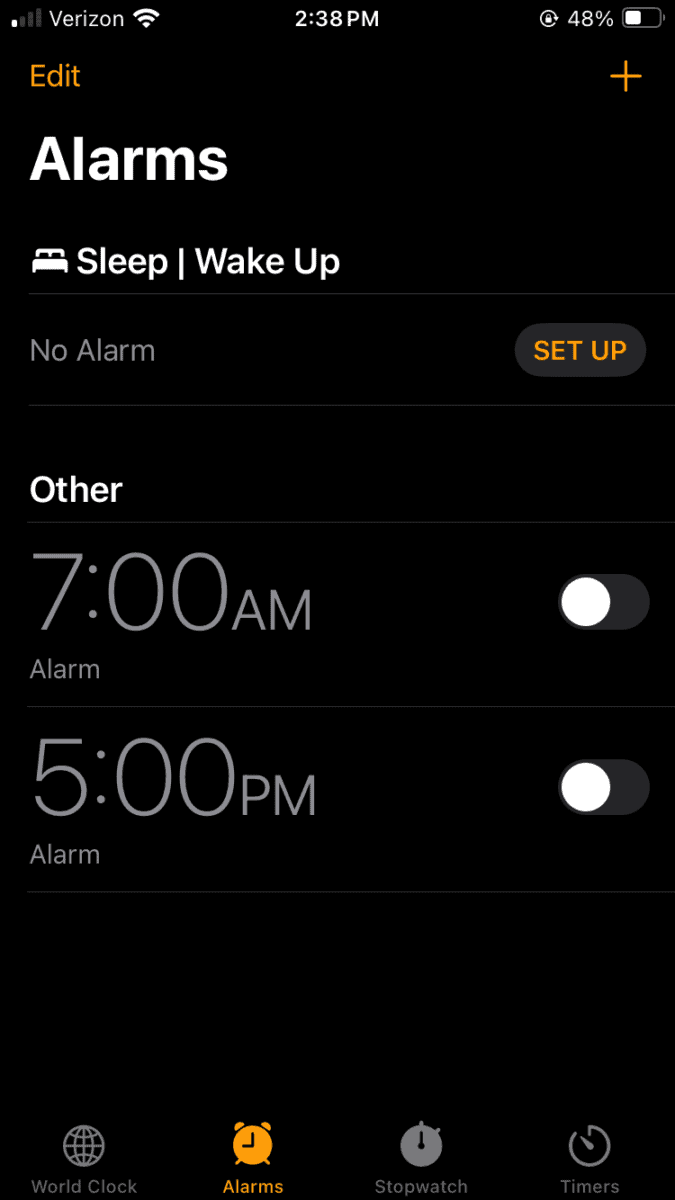The image displays a screenshot of a mobile device's alarm and clock application interface.

At the top, the status bar indicates "Verizon" as the carrier, with a Wi-Fi icon, the current time "2:38 PM," and a battery level at "48%." 

Below the status bar, the interface contains an "Edit" button on the left and an orange plus sign for adding a new alarm.

Dominating the screen is a large, bold white text that reads "Alarm." Beneath it, in smaller text accompanied by a bed icon, it says "Sleep | Wake Up." The status under this section indicates "No alarm" in grey text, with an "SET UP" button in orange capital letters below it.

Further down, another section labeled "OTHER" features two preset alarms:

1. "7:00 AM" is marked with a grey font and has an unactivated toggle switch to its right, indicated by being turned to the left. The word "Alarm" is written beneath this preset.
2. Similarly, "5:00 PM" is displayed with an unactivated toggle switch to its right, and the word "Alarm" below it.

At the very bottom of the screen, there are three icons: a globe icon labeled "World Clock," which is unselected; an orange-highlighted alarm clock icon labeled "Alarm," indicating the current section; and a clock icon labeled "Stopwatch."